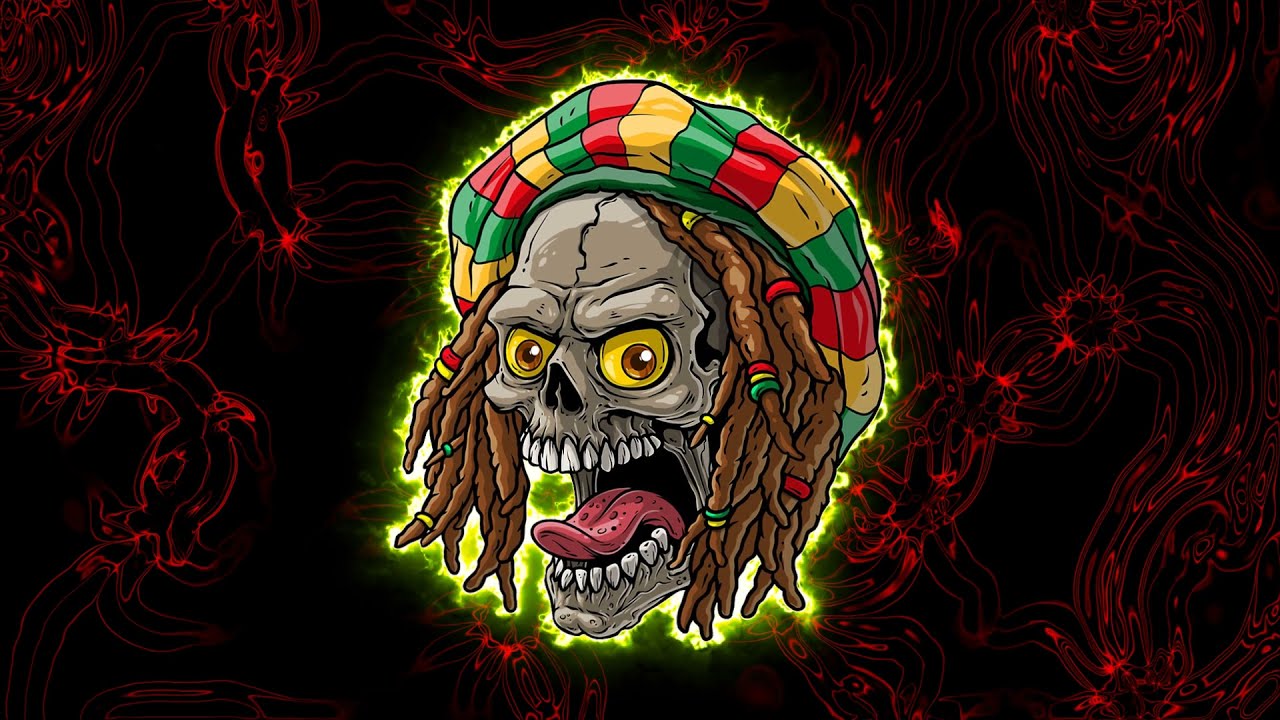The image depicts a computer-generated, animated-style horror scene focused on a ghastly skull with exaggerated features, likely intended for a horror movie or video game. The skull has bulging yellow eyes and an open mouth, where a pink tongue curls outward, as if it's exclaiming "blah." The skull has brown braided dreadlocks adorned with small red, yellow, and green bands. Topping off its head is a Rasta-style headscarf with matching red, yellow, and green stripes. The background is predominantly black, accentuated with red, vine-like lines or chains, rendering an eerie atmosphere. The entire skull has a faint yellow glow, adding to its terrifying appearance. Positioned centrally with no other focal objects, this unsettling image would likely be frightening for children.